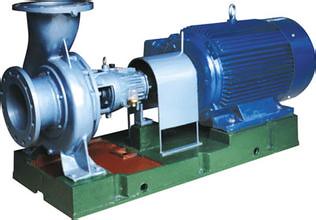The image depicts a detailed view of a mechanical assembly. The right side prominently features a cylindrical, blue metal component that appears to be an engine or a crucial part of a larger machine. This blue cylinder is intricately connected to another metallic component, which also exhibits cylindrical elements. The top section of the assembly seems designed for further connection to additional machinery, suggesting a modular construction. Both metallic parts rest on a green base, which also appears to be constructed of metal, indicating it's an integral part of the overall mechanism. The detailed interactions between these components highlight the complexity and precision involved in this machine's design.